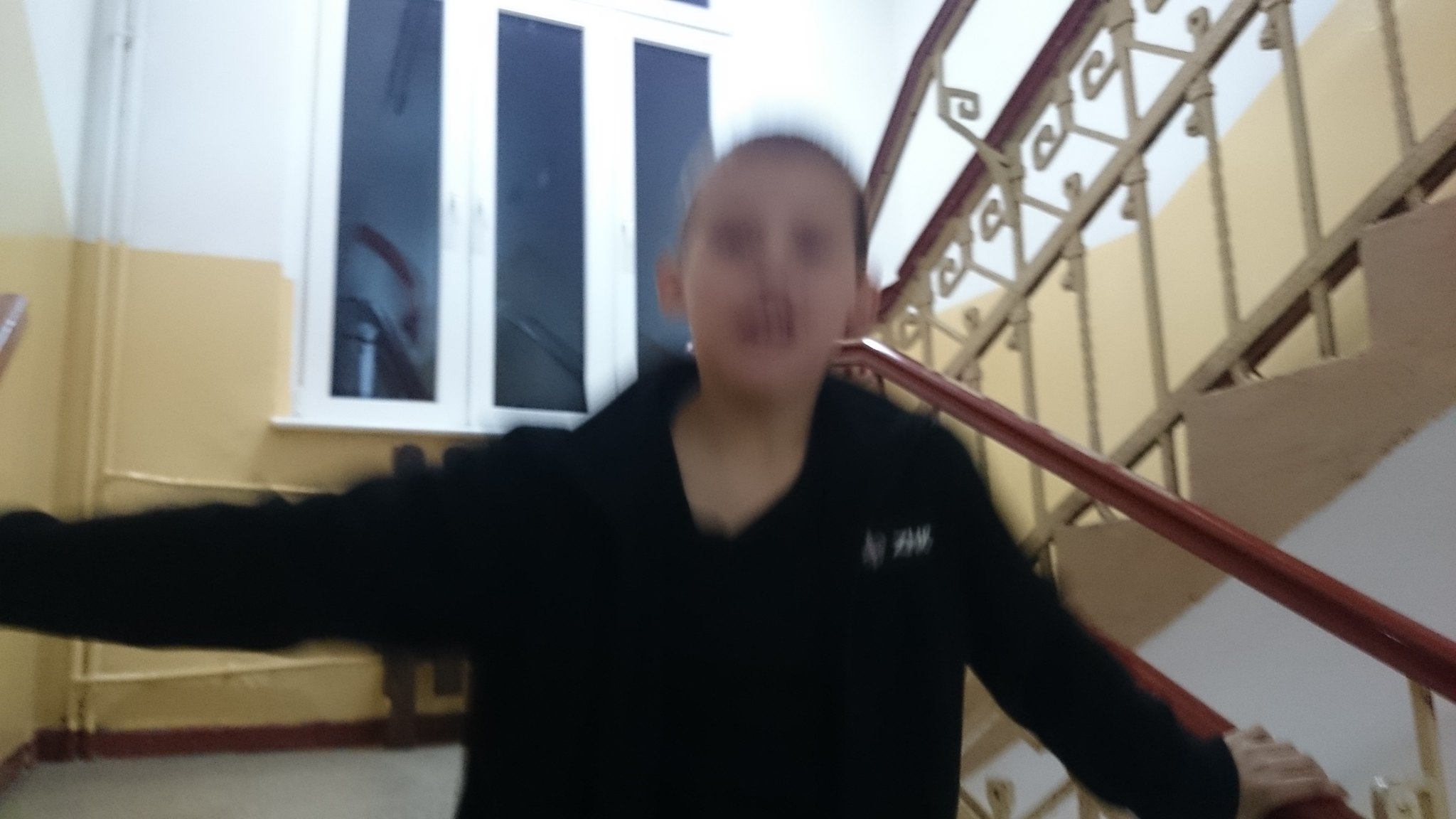In this photograph, a young child wearing a black sweater is captured midway through descending a stairwell. The child, who has cropped short hair, faces the camera with his left arm extended to grip a red railing on the right side of the image. His right arm stretches outward to the left, disappearing off-frame. Due to motion, his face is significantly blurred. The background features a distinct orange skirting along the base of a concrete wall that is painted yellow at the bottom half and white at the top. A window with three glass panels punctuates the wall, allowing light to filter into the stairwell. The stairs curve upwards to the right, featuring the continued red railing and vertical decorative railings adorned with a yellowish hue, providing a striking contrast to the otherwise muted tones of the setting.